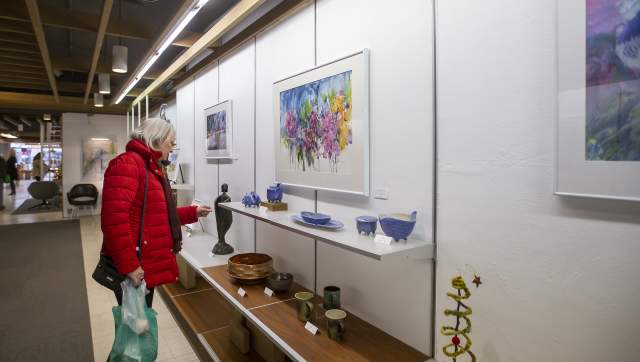In this image taken inside an art gallery or museum with white walls, a woman dressed in a red down jacket stands on the left side, holding a shopping bag in her right hand and a black purse slung over her shoulder. Her left hand is raised, reaching out to touch a small black statue shaped like a person that is displayed on a shelf. This shelf, located on the left, also holds various glazed plates and bowls. Below it, there is another shelf containing more art objects, including cups and a basket. The scene features multiple abstract paintings hanging on the wall, with one at eye level above the second shelf and others to its left and right. To the left side of the frame, light filters in from what appears to be the end of a hallway leading to the building's entrance. In the background, additional shelves and possibly some chairs are visible, illuminated by industrial ceiling lights. The woman appears to be the only person present in this thoughtfully curated space.